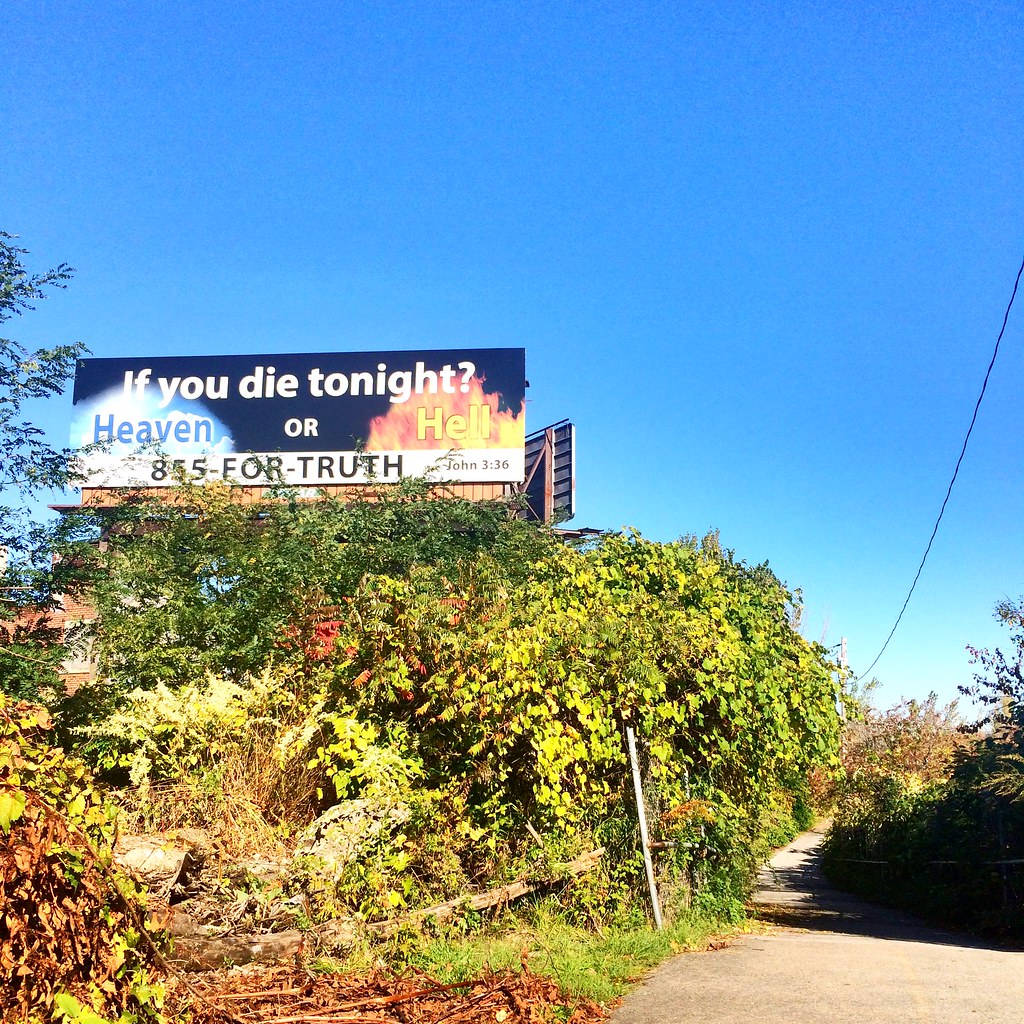A personal photograph taken during a sunny walk in the southern United States captures a vibrant blue sky occupying the upper half of the image. The lower half is divided into a trail on the right-hand side and dense brush and vegetation on the left. Among the foliage and trees, a prominent Christian-themed billboard stands out as the focal point. The billboard, with a navy blue background, features the message "If you die tonight" in white font. Below, the word "heaven" is in blue with an icy effect and a sunny, cloudy sky backdrop, while the word "hell" is in yellow with fiery imagery. Along the bottom of the billboard, a white bar displays the phone number "855-4-TRUTH" and a biblical reference, "John 3:36." Overhead, a cable line stretches across the scene. The mix of natural and constructed elements, along with the billboard's stark message, evokes a striking contrast in this detailed outdoor capture.